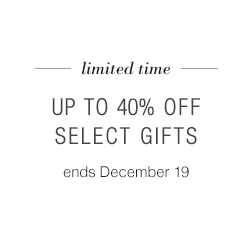The image features a promotional text snippet centered on a white background. At the very top, there are two solid lines flanking the phrase "limited time", which is italicized, bolded, in lowercase, and appears in a smaller font size compared to the rest of the text. Below this, in larger, all-capital letters and standard font, the message reads "UP TO 40% OFF SELECT GIFTS," with the "40%" represented numerically. This prominent offer is followed by another line of text stating "Ends December 19th," where the 'E' in "Ends" is lowercase, the 'D' in "December" is uppercase, and the date is expressed as "19." The spacing between these three distinct sections—the top promotional limit, the central discount offer, and the bottom end date—is uniform, adding to the centered and balanced appearance of the text.